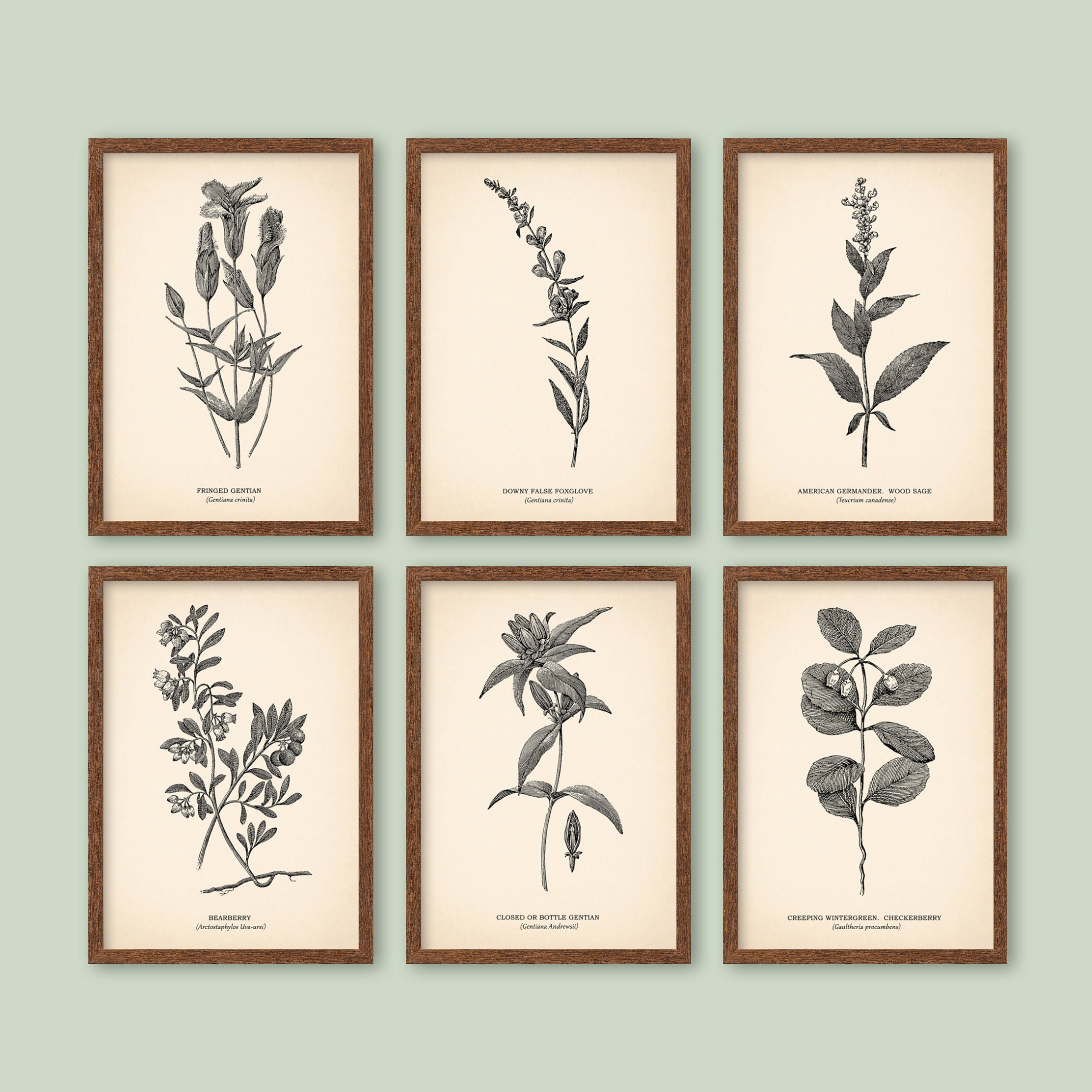This image features an intricately arranged art gallery display consisting of six framed illustrations, each meticulously hung in two rows of three on a light green wall. The artwork, likely computer-generated, appears vintage with black and white pencil drawings of various plants set against an off-white, cream-colored background. Each piece, approximately 11 by 17 inches, showcases different botanical specimens, accented with long stems and darker green hues suggesting dried foliage. Accompanying each illustration are barely legible names, from which only "Bearberry," "Fringed Gentian," and "Downy Falls Foxglow" can be discerned. The wooden frames add a rustic touch to the gallery, harmonizing with the overall subdued color scheme and enhancing the botanical theme of the display.